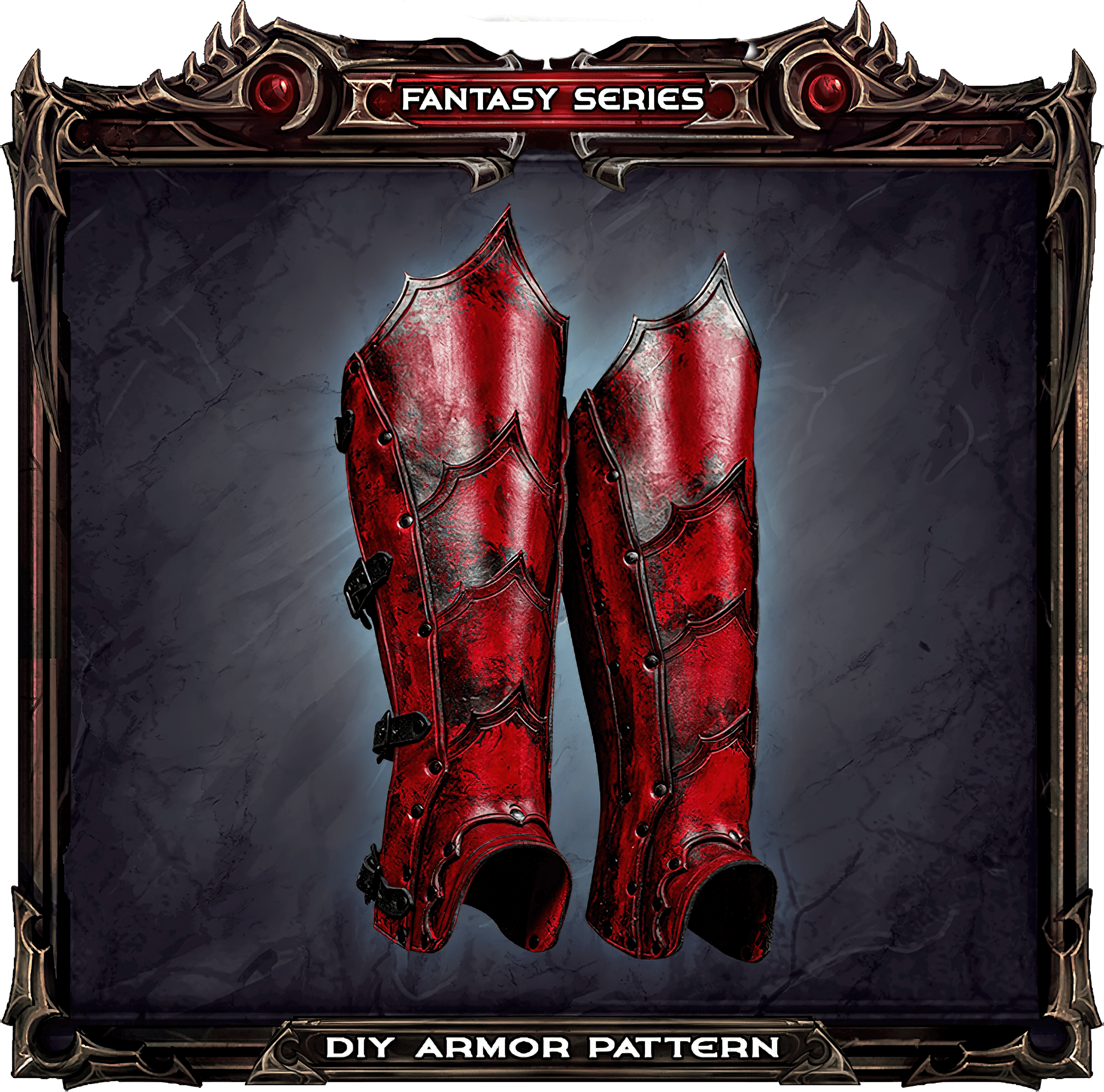This detailed image showcases a fantasy-themed, digitally crafted drawing of shin guards designed for cosplay, set against a blue background with a marbled black, white, and gray effect enhanced by a white highlight. The shin guards are elaborately styled, reminiscent of something from a Mad Max film with a gothic twist. They are predominantly red with brushed-on black accents to give a worn, medieval appearance. Featuring several segments riveted together, these shin guards also have spikes, black straps, and buckles for fastening. The frame surrounding the image is a thin, gothic-inspired border that enhances the rustic, metallic look. At the top, white text reads "Fantasy Series," while the bottom is labeled "DIY Armor Pattern," indicating a do-it-yourself approach to creating this striking piece of armor.